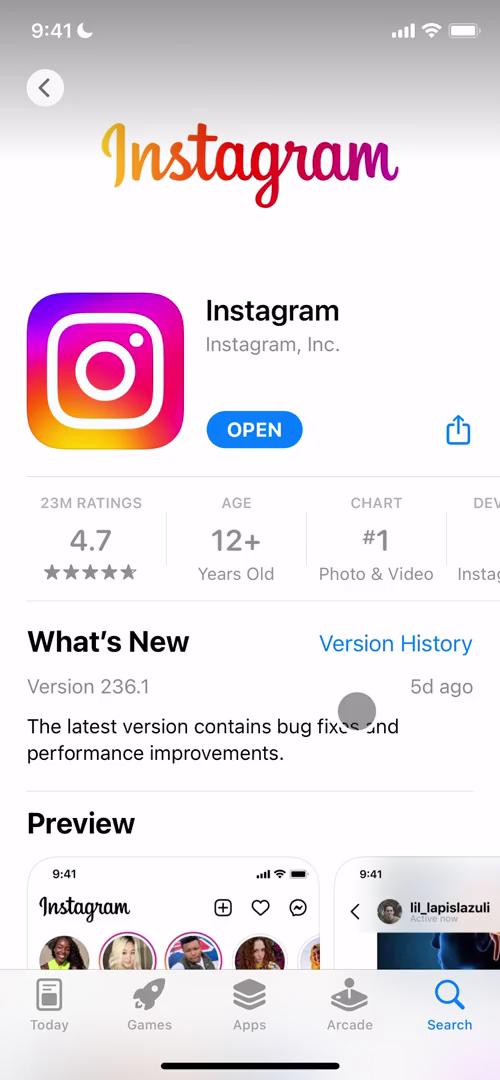This image is a mobile screenshot from the App Store, showcasing the Instagram app. At the top, the header displays "Instagram" in a cursive font with a gradient color scheme starting with light yellow and transitioning through orange, red, pink, and ending in purple. Below this header is the recognizably colorful Instagram logo—an icon resembling a camera—next to the name "Instagram" printed in a bold font. The app's publisher is noted with "Instagram, Inc." in gray text.

Next to the app information, there is a horizontal button labeled "Open," indicating that the app is already installed on the user's device. Beside this button is an icon for sharing the app. The layout is segmented by a series of gray dividers forming a structured grid. The first segment highlights "23 million ratings" accompanied by a 4.7 out of 5-star rating.

Following a small vertical line divider, the next section indicates the app's age rating of "12+ years old." Another subsequent vertical line notes the app's ranking: "#1 in Photo & Video." The next fragment appears to begin with "Dev," possibly short for developer information, but the text is truncated.

Proceeding downward, beneath another gray line, there is the section titled "What's New," with an adjacent link in blue labeled "Version History." The "What's New" text specifies that the current version is "236.1," and indicates that it was updated "5 days ago." The update notes detail that the "latest version contains bug fixes and performance improvements."

Another gray dividing line leads to the "Preview" section, showcasing multiple screenshots from the app. The bottom section of the screenshot features a navigation ribbon with five icons in gray. These represent different categories: "Today" (newspaper icon), "Games" (rocket ship icon), "Apps" (stacked books icon), "Arcade" (joystick icon), and "Search" (magnifying glass icon), with the "Search" tab highlighted in blue.